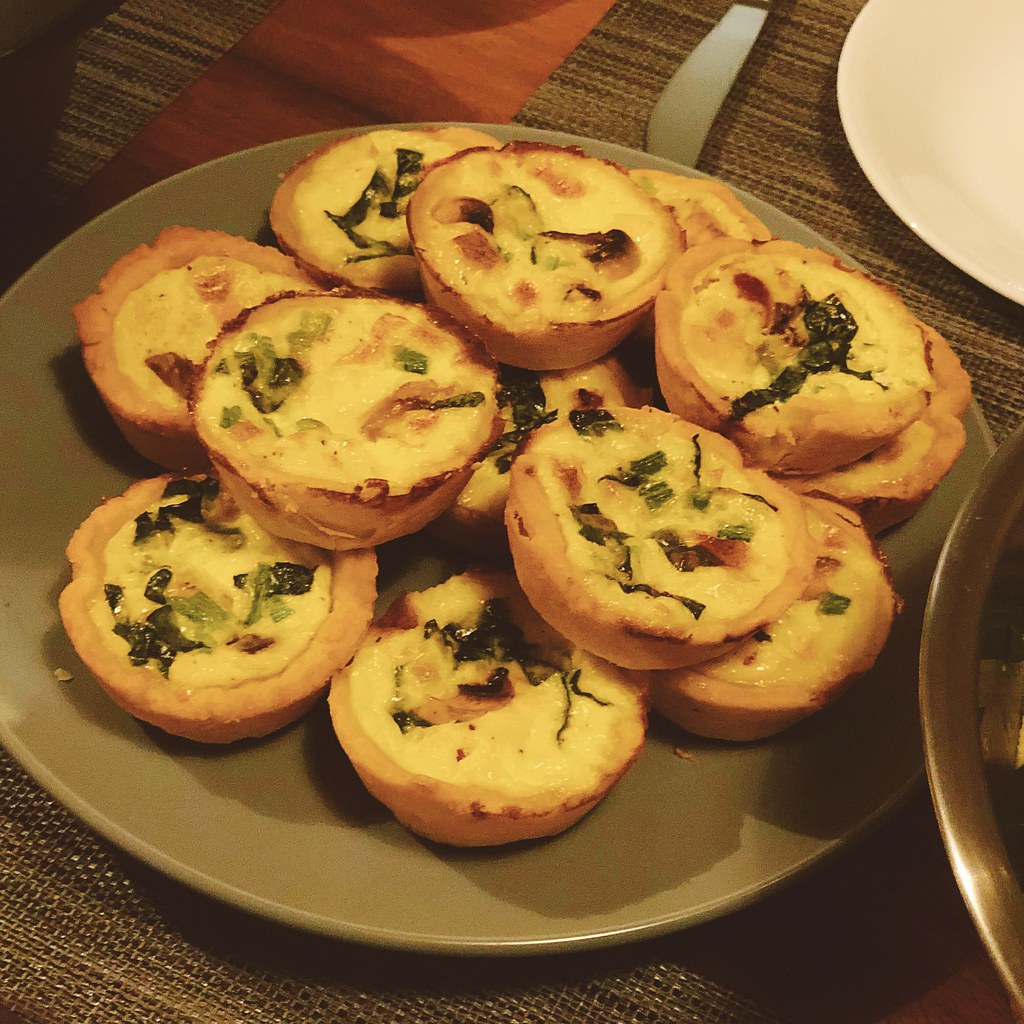The photograph showcases a beautifully arranged plate of food, highlighting a grayish gold ceramic dish that is filled with an enticing stack of mini egg quiches. These delightful bites are nestled in cup-shaped pastry shells that reveal a rich, yellow scrambled egg custard filling. Each mini quiche is studded with a colorful medley of vegetables, including greens, peppers, and possibly onions, adding a burst of flavor and visual appeal. The quiches exude a golden, baked hue, and are neatly stacked in two layers on the intricately woven, multi-toned brown placemat beneath. The detailed table setting includes a white round plate, a silver knife, and glimpses of a medium golden brown wooden table showing through the placemats. There's also a stainless steel bowl in the corner, enhancing the sophisticated restaurant-like atmosphere of the scene.